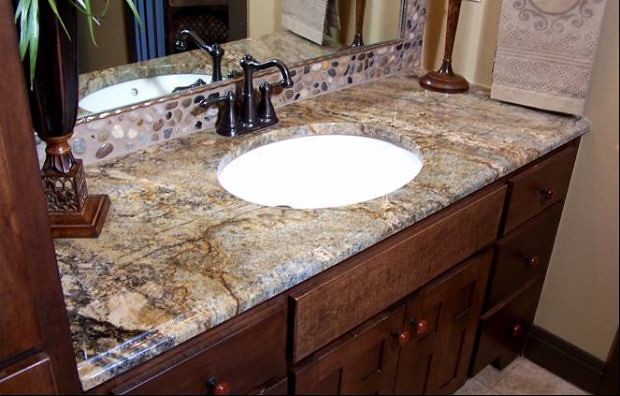A partial view of a bathroom showcases various elements and textures. To the left, a light brown wall serves as a backdrop. On the far wall, a beautifully patterned grayish-beige towel with swirls and circles hangs, adding an artistic touch. Dominating the scene is a large countertop with a sink, made of swirled marble in shades of brown, gray, and a hint of black. The faucet, a dark pewter color, stands out against the countertop. Above the sink is a wide mirror, reflecting a blue shower curtain and a nearby plant. On the counter are two distinct candlesticks, one with a wooden square base and the other with a tall, round base. The backsplash consists of stones set in concrete, featuring a mix of black and brown tones. Below, brown cabinets and drawers offer storage, and a tall shelving unit stands beside them, completing this detailed bathroom interior.